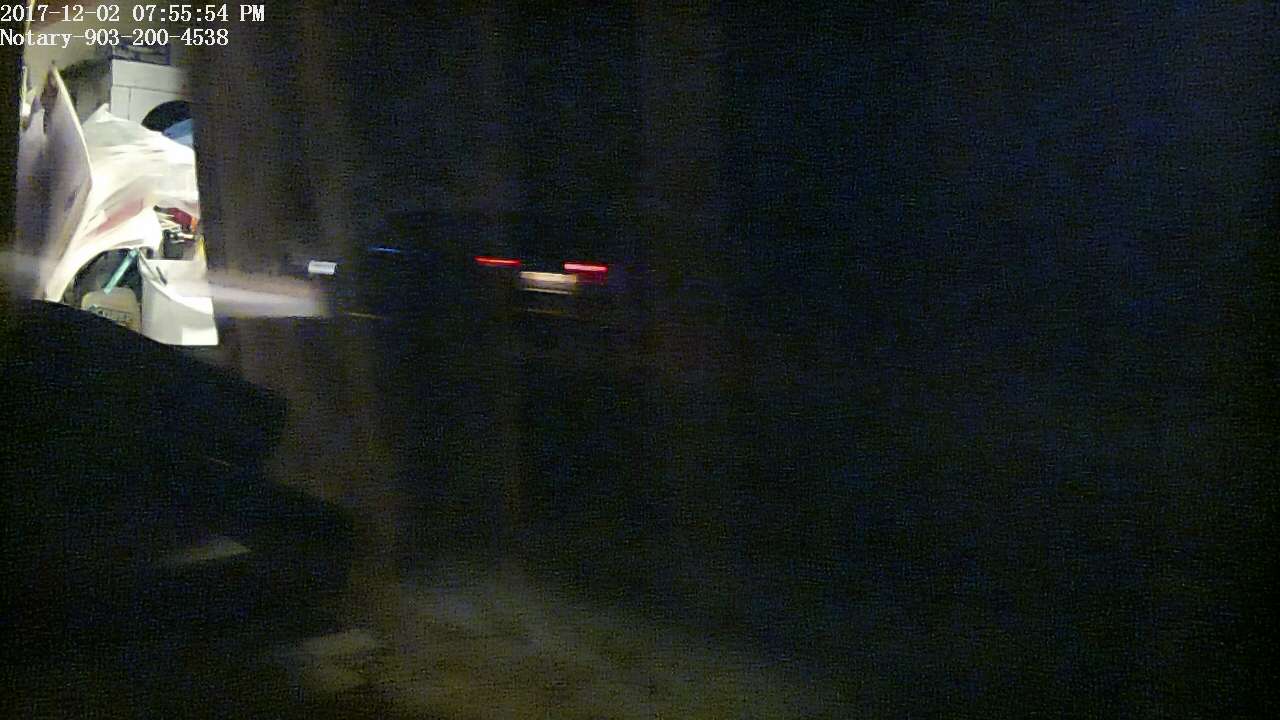A dim and blurred photograph with predominantly dark tones. The right half of the image is obscured in shadow, featuring vague doorway-like shapes and faint streaks resembling reflections of light. The left side is slightly more illuminated, showcasing a doorway with large, crumpled pieces of cloth or paper piled in front of what appears to be a washing machine or similar cabinet machinery. A dark, indistinct piece of furniture occupies the lower left corner. In the top left corner, a date and time stamp reads "2017-12-2, 755-54PM," followed by the notary's information, "903-200-4538."